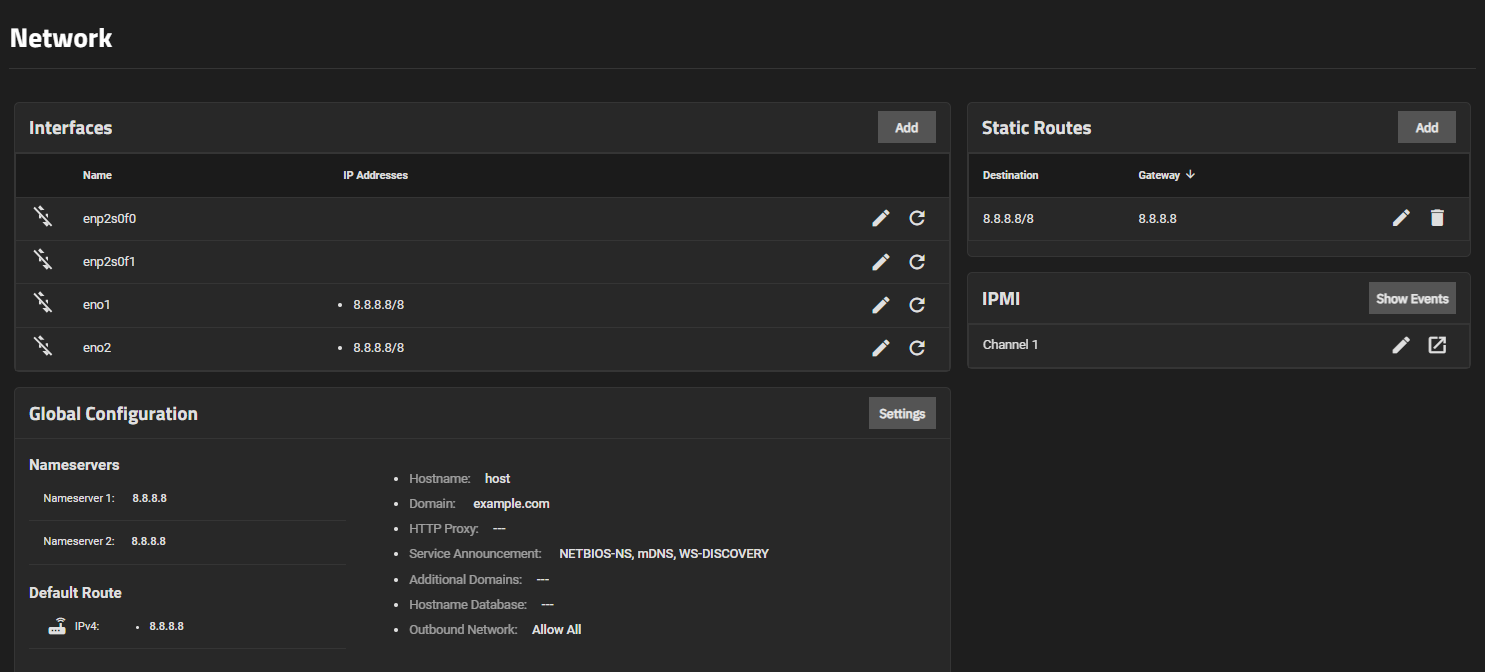This image captures the screen of a computer displaying a network interface management page. The page features a dark theme, with a black background and white text. In the top left corner, the words "Network" and "Interfaces" are prominently displayed on separate lines. At the far right end of the header, there is a grey button labeled "Add" in white text.

Below the header, there are sections titled "Name" and "Addresses." To the left of the names, which include identifiers like "NO1," "NO2," and "N2," identical icons resembling a line with dots on either side are present. The IP addresses field has mixed content; the first two rows are blank, followed by two entries displaying "8.8.8.8/8."

At the far right end of each row containing the names and IP addresses, there are clickable icons: a pen icon for editing and a refresh button for reloading the data.